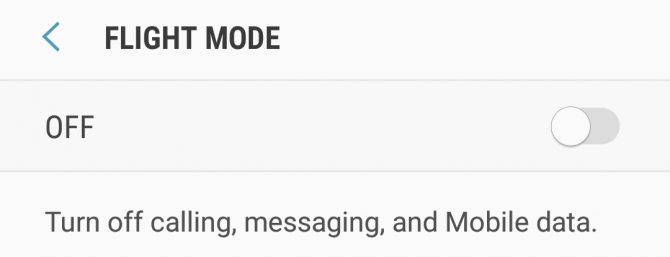**Image Description: Airplane Mode Interface on a Plain White Background**

The image features a minimalist user interface set against a plain white background, highlighting the 'Flight Mode' option commonly found on mobile devices. In the top portion, the term "Flight Mode" is displayed prominently in black block print, with a blue arrow pointing to the left of it. Below this text, a thin, faint blue line divides the screen.

In the lower section, a pale blue-bordered area is delineated by a darker blue line. Within this section lies a simple slider button interface, labeled "Off" in black print on the left side. The slider itself is a white button situated on a slightly darker blue background, currently positioned to the right, indicating that Flight Mode is turned off. 

Beneath the slider, black text provides a brief description: "Turn off calling, messaging, and mobile data," clearly explaining the function of Flight Mode. The overall design is straightforward, with no additional graphics or text, making it difficult to ascertain whether this interface belongs to an Android device or another operating system, as it appears even more streamlined compared to the Airplane Mode settings on an iPhone.